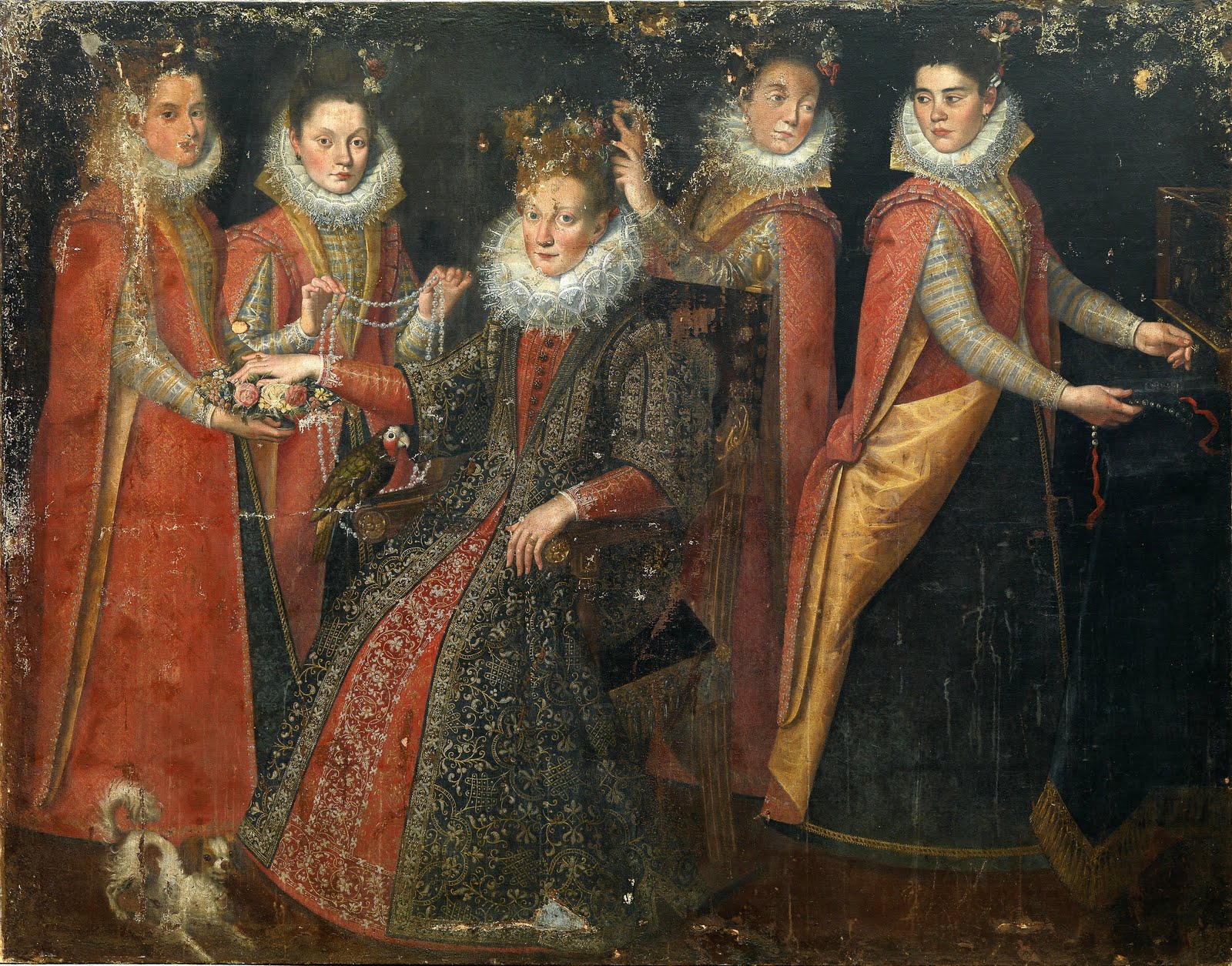This oil painting, which shows signs of age with some areas of peeling paint and slight creasing, depicts Queen Anne of England seated in the center, enveloped in regal elegance. She is adorned in a sumptuous red dress with a white ruffled collar and a black overcoat. Her strawberry blonde hair and rosy cheeks complement her fair skin. Around her, four ladies-in-waiting, dressed uniformly in red outfits with gold accents and matching ruffled collars, attend to her with meticulous care. To her left, one lady is either arranging the queen's hair or readying her crown, while another is presenting a pearl necklace for approval. Opposite them, another lady is possibly offering flowers or assisting with a spa-like treatment for her hands. In the right corner, a seamstress is seen attending to the queen's clothing. Adding a touch of charm, a small dog playfully crouches in the lower left corner, adding to the regal yet intimate atmosphere of this vintage European scene.